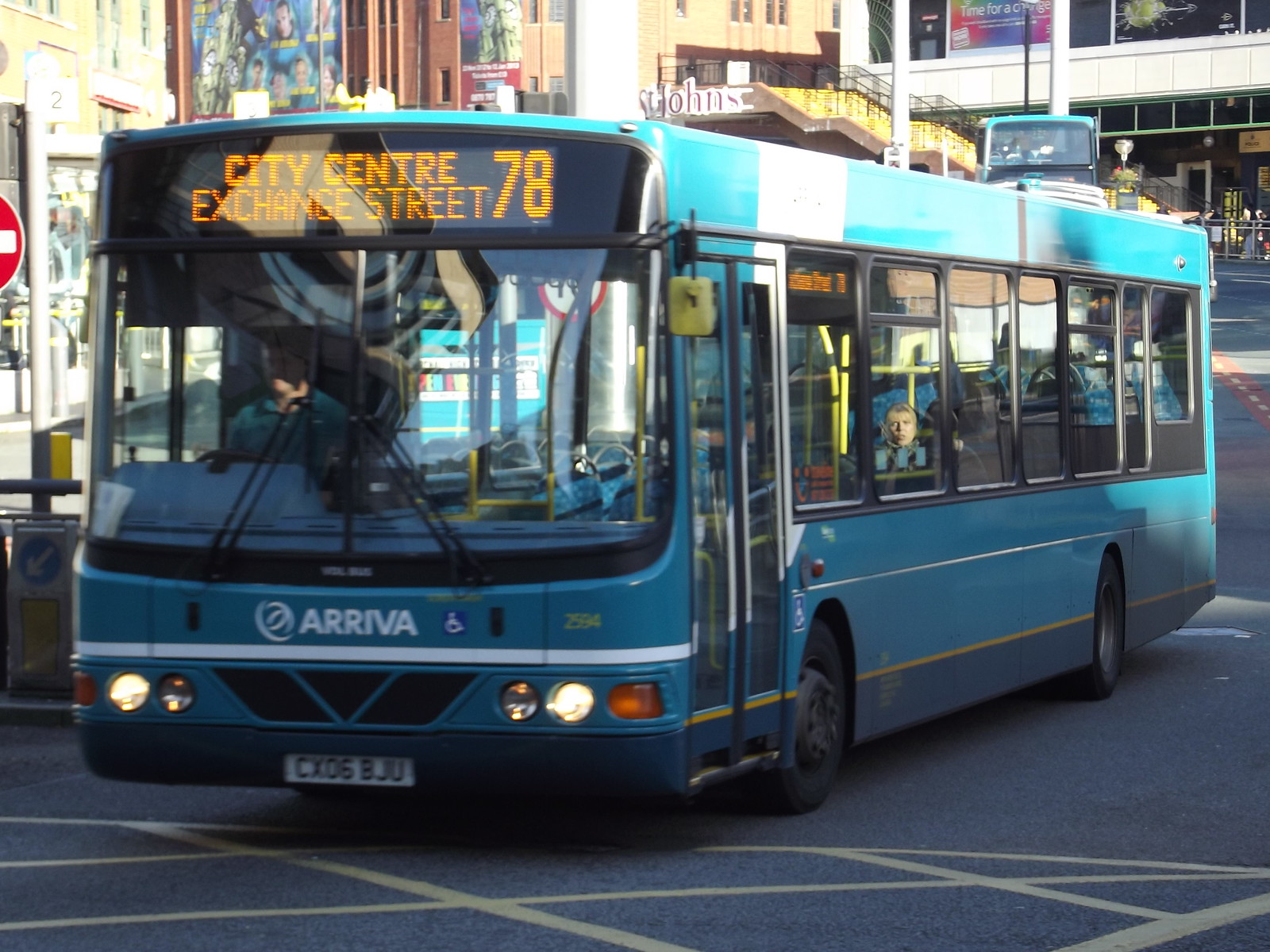This photograph captures an urban street scene in the United Kingdom, likely London, focusing on a city bus prominently positioned in the center of the frame. The bus, manufactured by Arriva, is painted in a striking combination of teal and dark blue, separated by a yellow line. The destination is displayed on a digital banner above the driver's compartment, reading "City Centre Exchange Street 78," a detail further supported by the British spelling of "Centre." The bus bears the license plate CX-06-BJU, a format consistent with European standards.

The bus's exterior features essential details such as the Arriva logo in white and an accessibility logo for handicapped passengers, accompanied by the number 2594 in yellow. The vehicle has two illuminated round headlights at the front. Notably, the driver's seat is on the left side, adhering to British driving conventions. 

In the image, a reflection of a man is visible in one of the windows, though there is also a woman passenger looking directly at the camera, indicating the bus is not entirely empty. The background includes urban architecture with multiple buildings, one of which is identified as "St. John's." The bus is captured at a crosswalk denoted by yellow crisscrossing stripes, adding to the scene's metropolitan character. 

Overall, this detailed photograph not only highlights the distinctive features of the Arriva city bus but also vividly captures its urban setting within the United Kingdom.